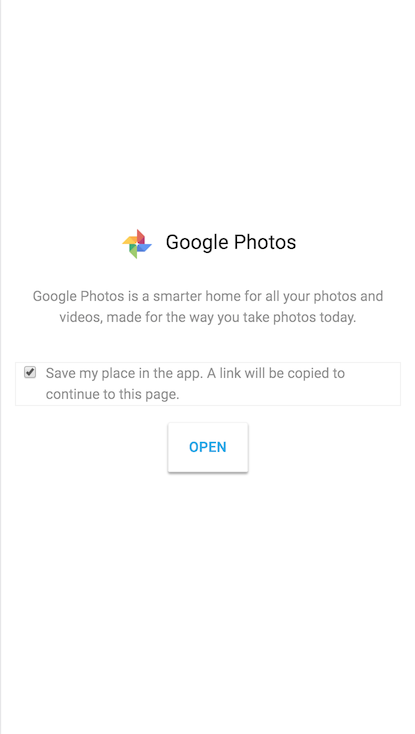The image depicts the initial setup page of the Google Photos app. Dominating the center of a white background is the colorful Google Photos icon, featuring the hallmark colors of yellow, red, blue, and green. Directly below the icon is the text "Google Photos" rendered in black. 

Beneath the app name, a brief description reads: "Google Photos is a smarter home for all your photos and videos, made for the way you take photos today." Further down, there's an option accompanied by a checkbox labeled: "Save my place in the app. A link will be copied to continue to this page." This box is ticked, indicating user consent. 

A prominent blue button labeled "Open" sits at the bottom, inviting the user to proceed. The overall design is minimalist, with ample white space and gray text, making the colorful icon and the blue button stand out. This screen is likely presented to users when they first open the app or when setting it up on a new device.